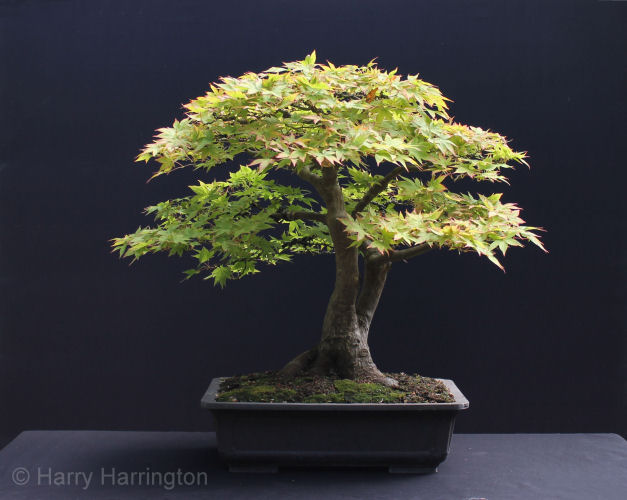This detailed image portrays a beautifully shaped bonsai tree growing from a low, rectangular, gray planter. The planter is filled with visible soil and vibrant green moss, adding to the aesthetic appeal. The bonsai features two main trunks that diverge at the base, providing an elegant, natural split leading upwards into branches. These branches are adorned with numerous small, green leaves, showcasing the careful cultivation of the tree. The photograph has a predominantly dark blue backdrop that enhances the bonsai's delicate form and is complemented by a dark blue surface below. An artificial light source illuminates the scene from above, highlighting the tree's intricate details. Additionally, the image bears a copyright mark at the bottom that reads "Harry Harrington," adding an artistic touch to the presentation of this serene bonsai tree.